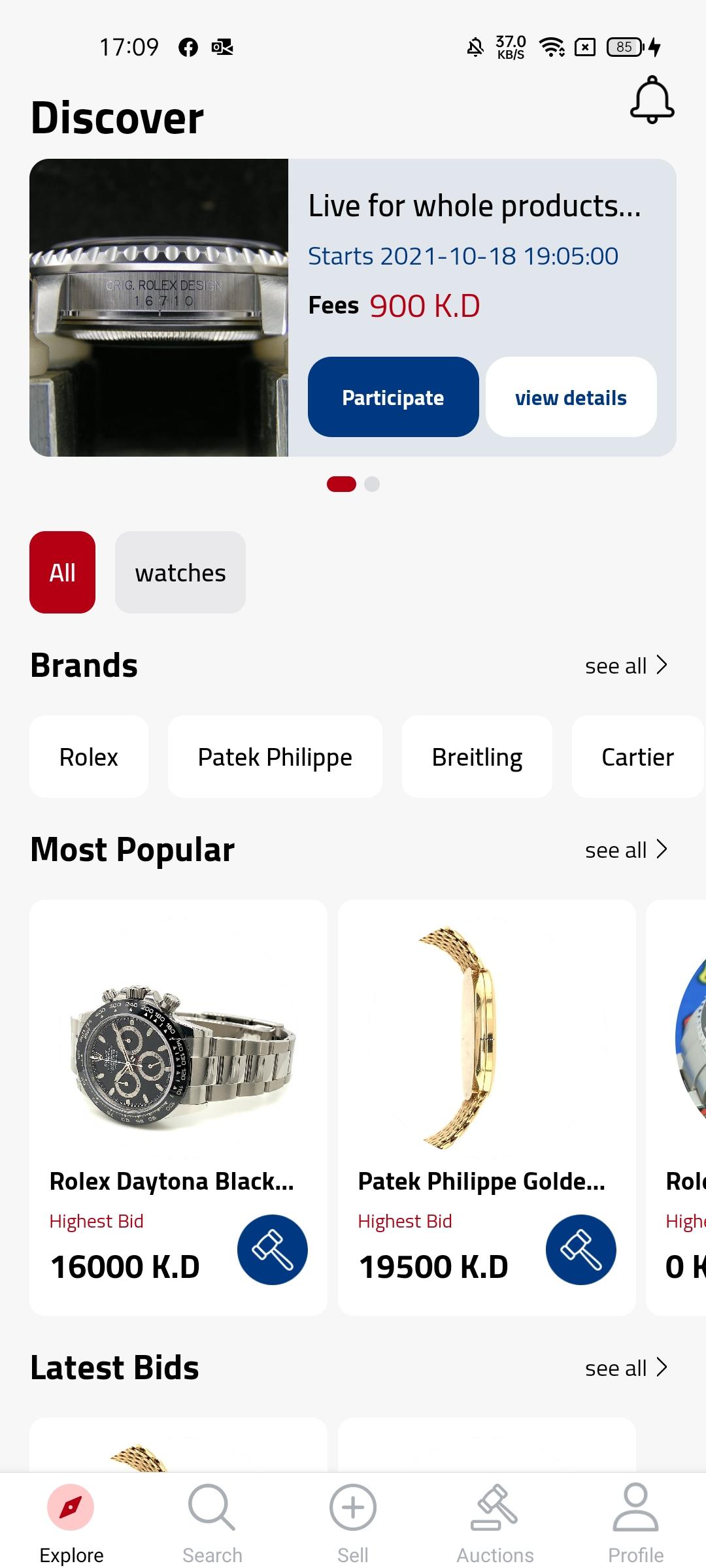This image depicts a mobile app interface for purchasing watches. In the top left corner, the word "Discover" is prominently displayed. Below it is a section highlighting a product with an accompanying image of a watch. The caption for this product reads, "Live for a Whole Products," with a start date of 2021-10-18 and a price beginning at $19.05. Additional details mention the terms "free" and "900KD." Beneath this information, there are two interactable buttons labeled "Participate" and "View Details."

To the right of this section, there is a close-up image of the side of a Rolex watch, showcasing intricate details, including part of the watch face and a metal plate. Another section below features a list of the most popular items. It includes images and details of two luxurious watches: a Rolex and a Patek Philippe Golden Watch. The Golden Watch is priced at an impressive $19,500KD.